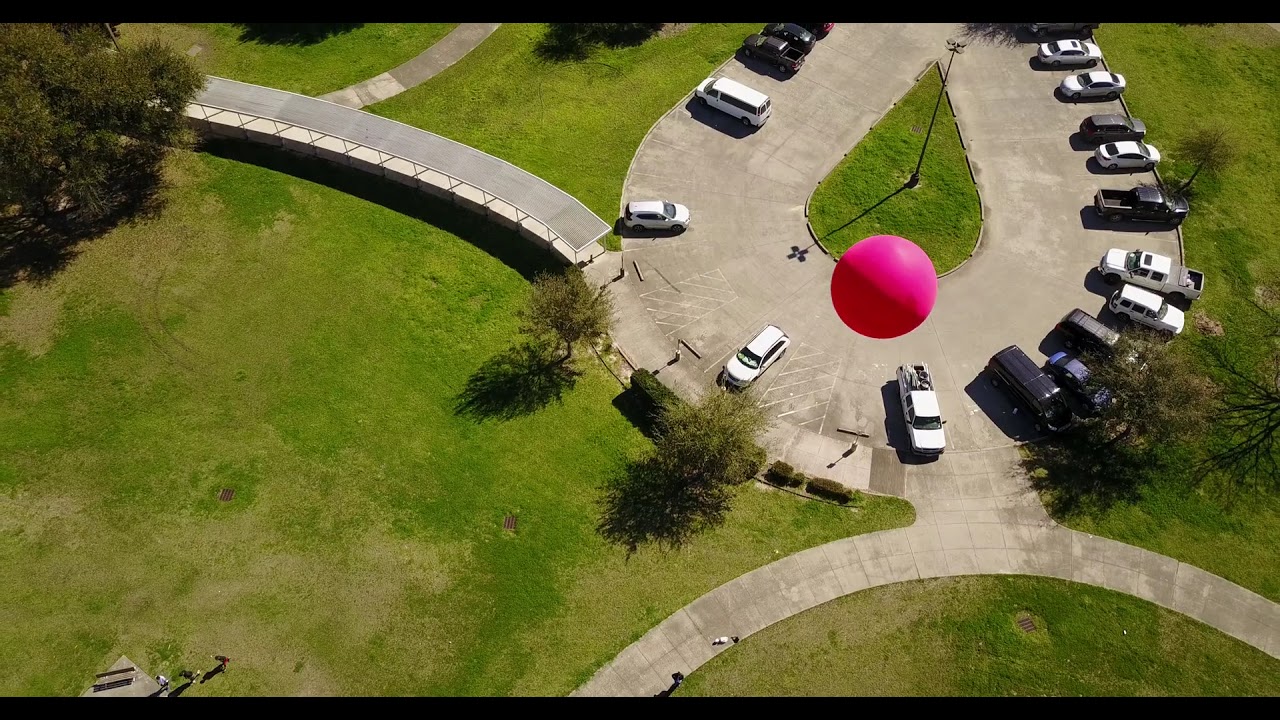The image is an aerial photograph of an outdoor park area with a teardrop-shaped parking lot located on the right side. The parking spaces are arranged around the edges of the teardrop shape, and several white trucks and cars are parked, with a few spaces remaining open. At the center of the teardrop is a conspicuous, unnatural-looking pink circle that appears digitally added to the image. Surrounding the parking area is a well-maintained grassy surface, with trees visible in the top left, center, and off to the right side of the image.

Connectivity to the parking lot appears limited, as the only visible path to it is a pedestrian walkway on the lower right, which looks too narrow for vehicular access. There might be another entrance not visible in the image. Additionally, there is a covered walkway with a gray roof extending from the left side of the parking area towards the upper left. The scene is set outdoors during daylight, with a palette of green, yellow, brown, gray, pink, white, and red colors. The overall setting suggests a serene park space integrated with limited parking facilities.